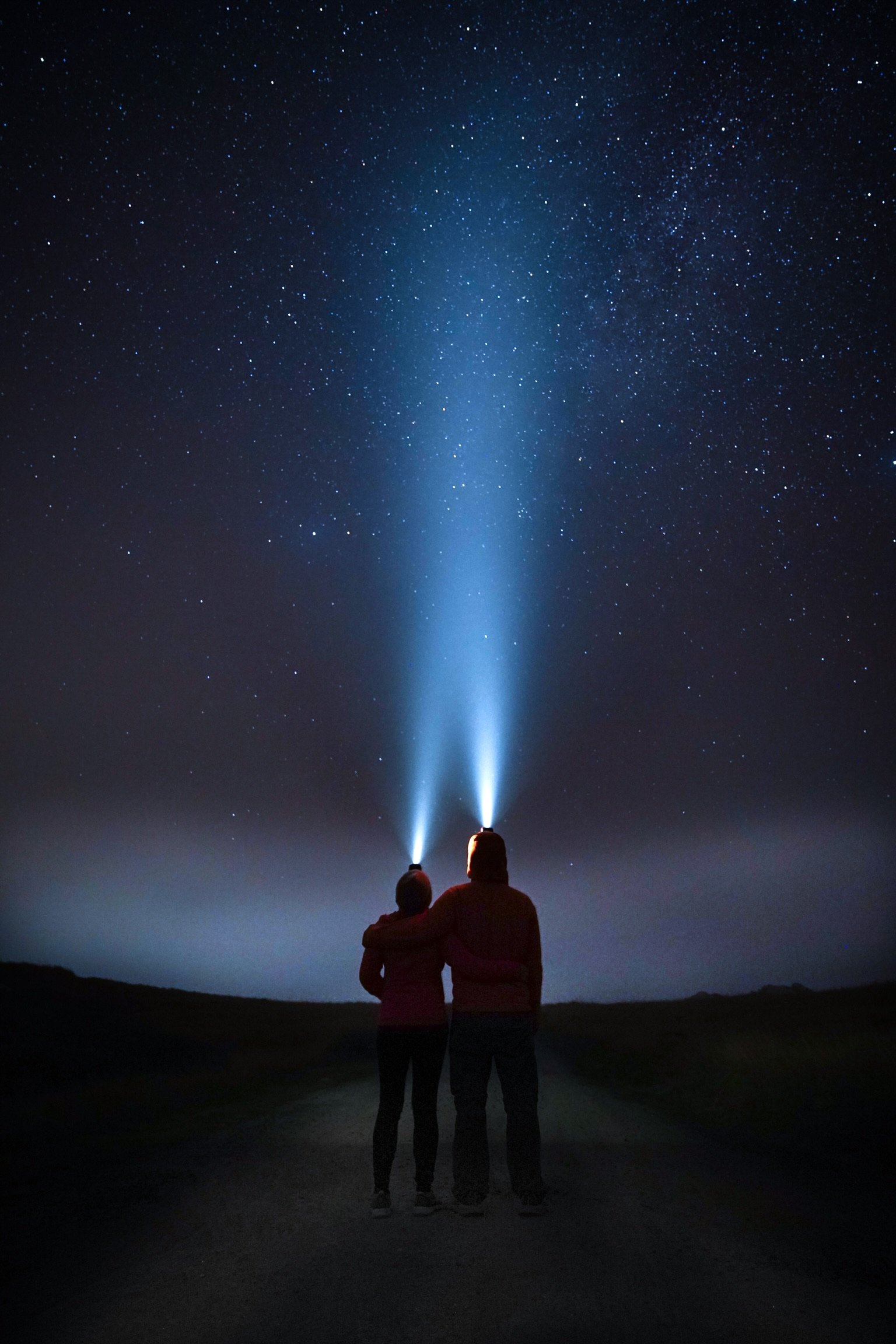Against a backdrop of a magnificent, starry night sky transitioning from deep blue at the horizon to an almost inky darkness above, a couple stands close together on a pathway or road. The dark surroundings give little geographic indication of their location, save for the faint outline of a hill or plant life. The night is clear with minimal clouds and the sky is awash with countless stars, punctuated by a slight haze along the horizon suggestive of distant city lights.

The couple is clad in winter attire: dark pants and puffer jackets in shades of red and orange. Each wears a headlamp that emits a strong beam of light, dramatically illuminating the night sky above them. The taller figure, likely a man, has one arm affectionately draped over the shoulders of the smaller figure, presumably a woman, who has her arm around his waist. Both figures gaze upward, their headlamps creating twin pillars of light reaching towards the heavens, as they share a moment of awe under the beautifully star-studded night.